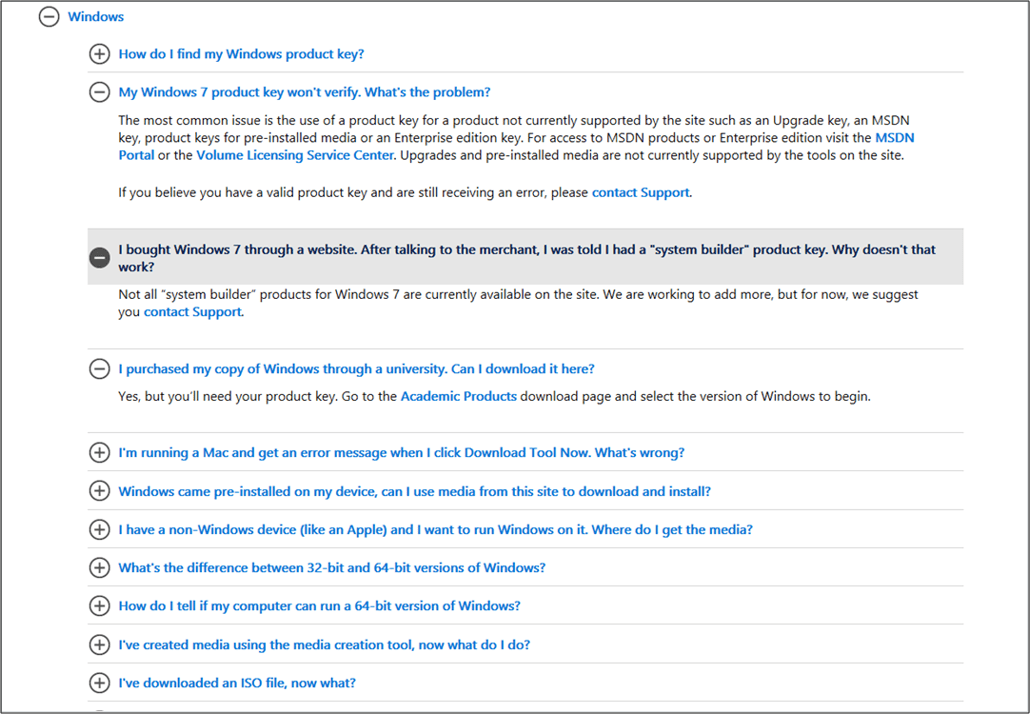The image is a screenshot of a Microsoft Frequently Asked Questions (FAQ) page, designed in a classic informational format. The layout of the image is wider than it is tall, approximately by a ratio of 30%. It features a clean white background with a thin black line framing the outer edge.

At the top of the image, there is a parent navigation menu indicated by a circle with a black minus sign in the upper left corner, next to the word "Windows" in blue, suggesting it is a clickable link. This menu structure proposes a hierarchical drop-down design common to FAQ sections.

Indented below the parent menu, the first item begins with a plus sign inside a circle, followed by the question "How do I find my Windows product key?" in blue text, indicating that this section is collapsible and currently unexpanded.

Further down, the expanded section is identified by a minus sign and contains the question "My Windows 7 product key won't verify. What's the problem?" in blue text. Beneath this, there is a paragraph providing the solution or explanation for this particular issue.

Another expanded section follows, highlighted with a gray background for distinction. It begins with a circle featuring a black background minus sign, while the question "I bought Windows 7 through a website after talking to the merchant. I was told I had a system builder product key. Why doesn't that work?" is displayed in dark blue text. This reverse color scheme emphasizes this particular query. 

The detailed information and visually organized queries on this FAQ page are typical of a streamlined user support interface, aimed at effectively aiding users in troubleshooting common issues.